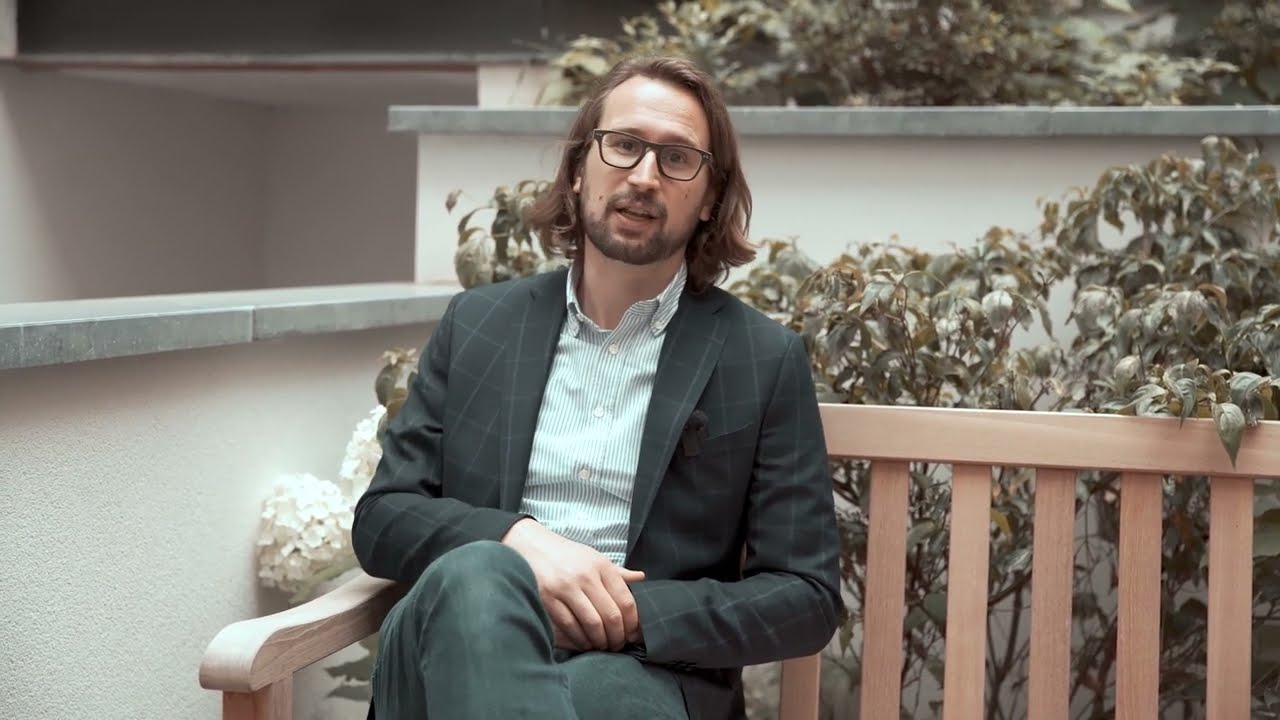A man likely in his 30s with a brown beard and long brown hair, tied to the length of his leg, sits on a wooden bench with vertical cutouts on its backrest. He wears black-rimmed glasses and is dressed in a distinct outfit: a black blazer with a fine white grid-like pattern, a red shirt underneath, and black pants. The setting appears to be outdoors, possibly on a college campus, as suggested by the maintained shrubbery and plants surrounding him. Behind the bench is a white wall with a stone ledge on top, and a variety of green plants rise above it. The overall atmosphere is one of a serene, well-kept environment, akin to a landscaped public or academic space.